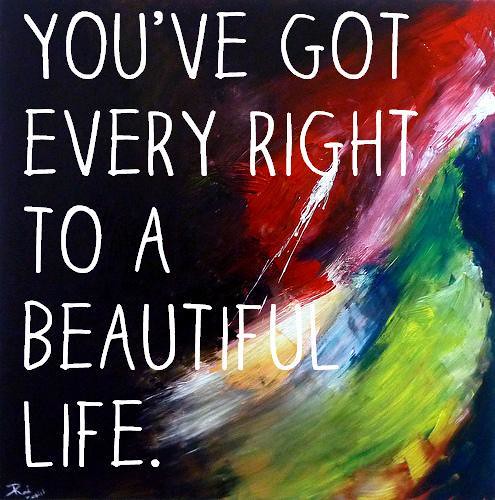This square image features an abstract piece of artwork that combines dark and vibrant colors. The left side is predominantly dark, transitioning from a deep blue to almost black, with hints of purple. On the right side, there's an array of colorful paintbrush strokes blending together. At the top right, the colors are mainly red and dark purple, intersected by a pink stripe that runs downward where the red meets a green portion extending to the bottom right. Near the edge of the green area, there's yellow and brown smudges, with a distinct blue spot in the center. Overlaying this backdrop, in large, all-capital white letters from the top to the bottom, is the quote, "YOU'VE GOT EVERY RIGHT TO A BEAUTIFUL LIFE." In the bottom left corner, a tiny white signature appears, which begins with an "R" but is otherwise indistinct.